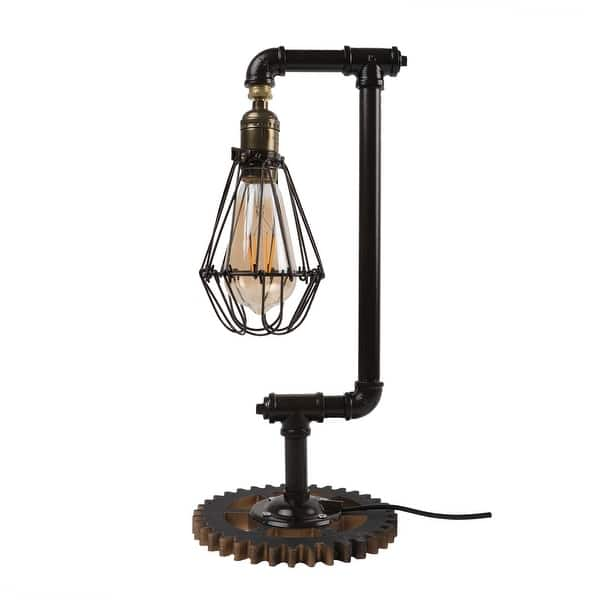This image features a distinctive lamp designed with a steampunk aesthetic. The base of the lamp is crafted from a large gear, likely repurposed from heavy machinery, featuring prominent teeth. Attached to the gear is a black circular platform, from which a short black metal pipe extends vertically. This pipe, resembling a water pipe that's been spray-painted black, connects to a three-way connector about five inches up. From there, the pipe takes a series of right and left 90-degree turns, creating a unique, geometric framework.

The light bulb is housed in a caged container, made from black metal wire, further emphasizing its industrial look. The lamp’s design includes needle-like points around the cage, adding to its modern and new-age appeal. The light bulb itself emits a yellow-orange glow, enhancing the overall steampunk vibe. The simplicity of the white background contrasts with the intricate metalwork, highlighting the lamp's unique construction and aesthetic.